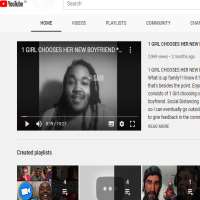Here is a detailed and cleaned-up description of the screenshot:

---

The image captures a small section of a YouTube interface. It features a white background with the YouTube logo positioned in the upper left corner. The logo comprises a red square with a play button symbol (a yellow or white triangle pointing right) that is hard to discern due to the text size. To the right of the logo, "YouTube" is clearly visible, followed by some additional text indicating a regional or subsidiary version of the site, such as YouTube UK or YouTube Colombia.

Below this, there's a white search bar containing the greyed-out text "Search." Directly beneath the search bar is a menu with a darker grey background. The "Home" option is highlighted in black and underlined to indicate the current active page. Next to "Home," in grey text, are additional menu options: "Playlists," "Community," and another partially visible option.

Further down the image is a video in 4:3 aspect ratio, resulting in black bars on either side. The video appears to be a few seconds into playback. The title at the top reads "One Girl Chooses Her New Boyfriend." At the bottom of the video frame, standard playback controls are visible, including the play button, volume control, elapsed time, closed captions, and the settings gear icon.

On the right side of the video, there is some black text, although it is unclear what it says. The lower portion of the image features thumbnails of recommended videos, which appear to be of low quality or outdated content.

---

This description provides a detailed and organized overview of all the elements visible in the screenshot, accurately conveying the information given in the original voice caption.